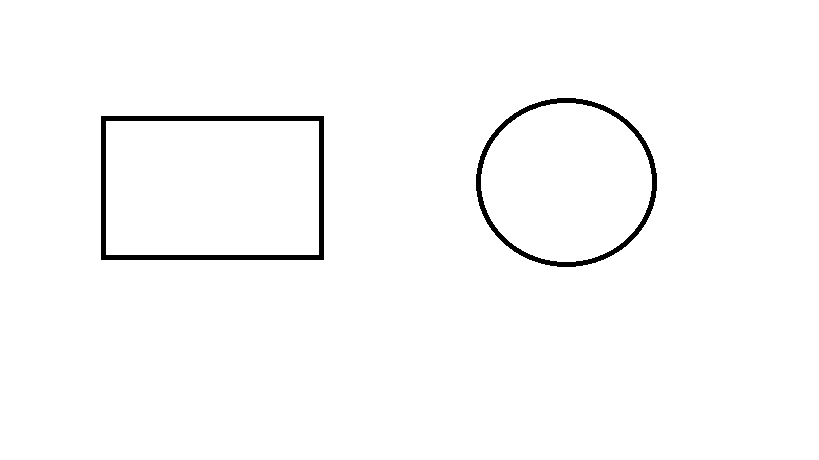This black and white line drawing, likely computer-generated and somewhat pixelated, features two distinct geometric shapes against a completely white background. The shape on the left is a rectangle, approximately 40% wider than it is tall, making it a horizontally oriented, thin black line with perfectly straight lines and 90-degree corners. The interior of the rectangle is white, and it is outlined by a single, continuous black line.

To the right of the rectangle is an oval, which stands slightly taller than the rectangle but is not as wide. This oval appears to have been a circle that has been horizontally stretched by about 15%. Like the rectangle, the oval is outlined by a single black line of a similar width. 

Both shapes are vertically aligned along their central axes, with the oval being marginally taller than the rectangle. The simplicity of the design, combined with the precise geometry of the shapes, creates a minimalist composition that draws attention to the stark contrast between the black lines and the white background.